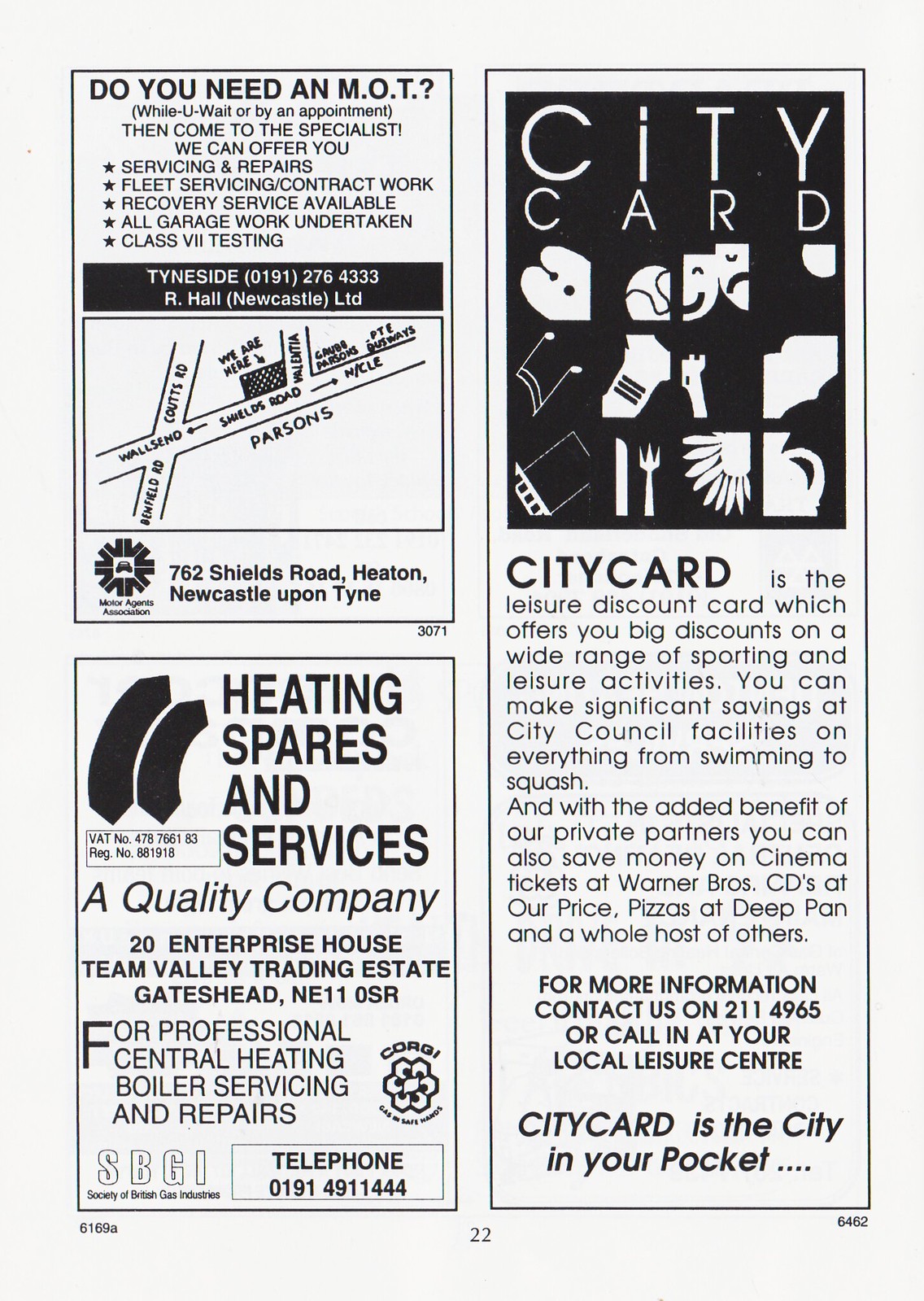The vertically aligned rectangular image features a white sheet of paper, indicating page number 22 at the bottom center. It comprises three distinct advertisements, each framed in black rectangular sections. 

In the upper left-hand corner, the first ad is labeled "Do you need an MOT?" and offers services such as servicing, repairs, fleet servicing, and contract work. This section includes bullet points shaped like stars, a contact name, a telephone number, and a small black-and-white map pinpointing the address: 762 Shields Road, Heaton, Newcastle upon Tyne.

Below this, the second ad is titled "Heating Spares and Services" in bold black letters, branding itself as "a quality company." It promotes professional central heating, boiler servicing, and repairs, providing contact information at the bottom.

The entire right side of the page is occupied by a large advertisement for "City Card" in bold black letters. This ad highlights City Card as a leisure discount card and elaborates on benefits such as significant discounts on various activities city-wide. It concludes with the slogan "City Card is the city in your pocket," along with additional contact information.

The layout resembles clipped newspaper advertisements, meticulously organized into these three sections, offering a range of services from vehicle maintenance to home heating solutions and leisure activity discounts.